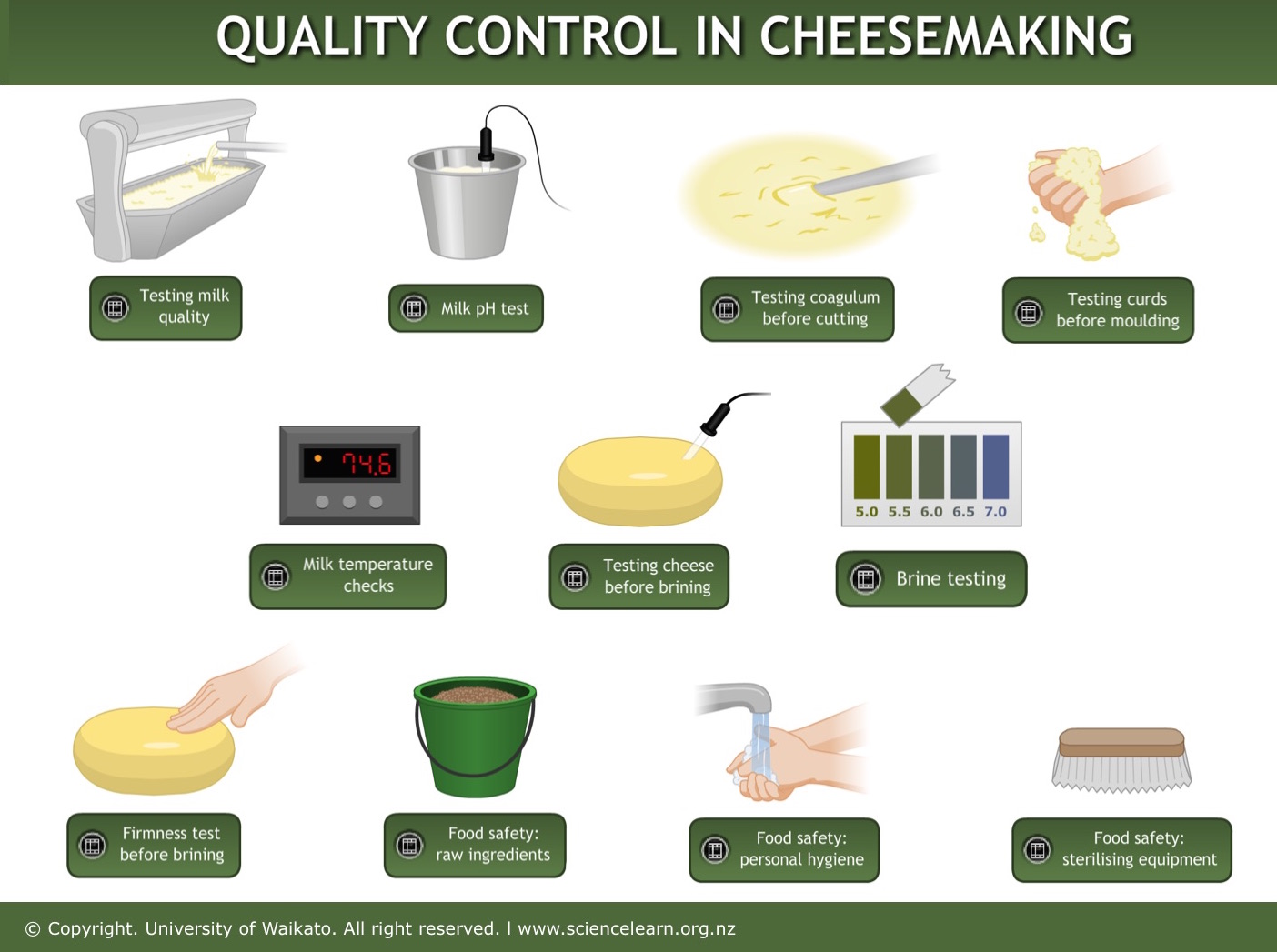The image features a white background and a prominent green box at the top with the white text "Quality Control in Cheesemaking." It is divided into multiple sections, each illustrating different steps and equipment used in the cheesemaking quality control process. The first section shows a metallic vat with a green label beneath it that reads "Testing Milk Quality." Next, a bucket with a corded device, labeled "Milk pH Test," is depicted. Following that, there's an illustration of a spoonful of thickened batter captioned "Testing Coagulum Before Cutting," and an image of curds being held, labeled "Testing Curds Before Molding."

The subsequent row portrays "Milk Temperature Checks" alongside a digital clock, "Testing Cheese Before Brining" with a piece of cheese, and a brine pH testing kit. Further down, the illustrations include "Firmness Test Before Brining," "Food Safety Raw Ingredients," "Food Safety Personal Hygiene," and "Food Safety Sterilizing Equipment."

At the bottom, a green rectangle displays the copyright notice: "University of Waikato. All rights reserved," along with the URL www.sciencelearn.org.nz. The illustrations are cartoonish in style, providing a clear, visual guide to the methods and equipment necessary for quality control in cheesemaking.